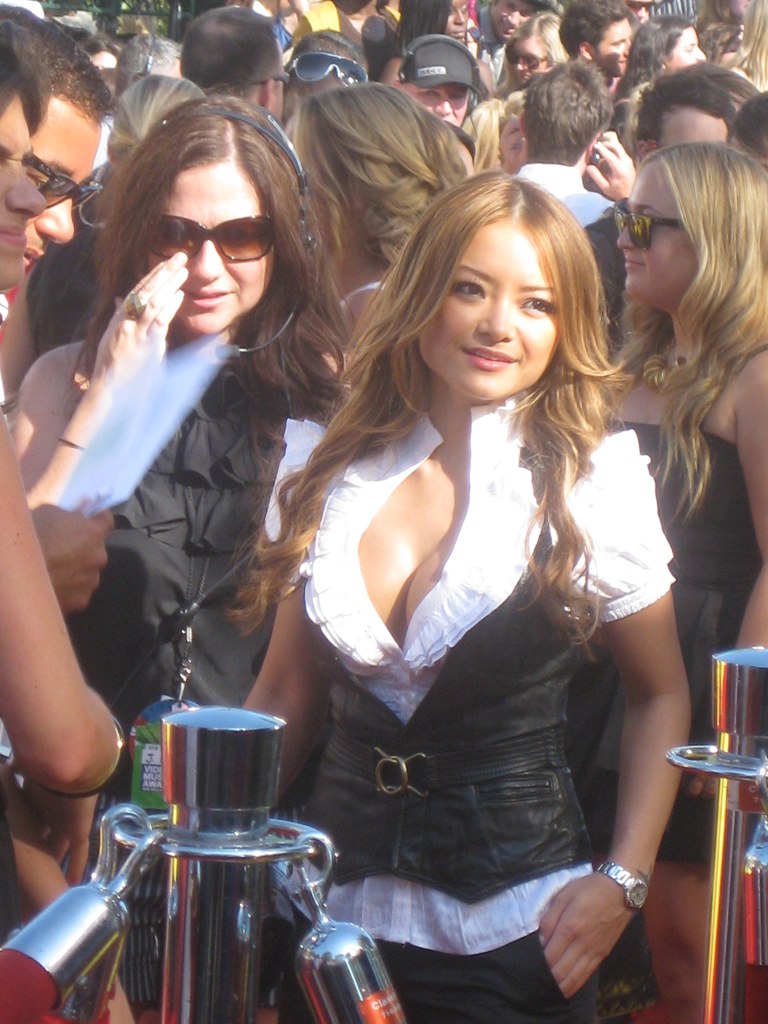The image captures a bustling event, reminiscent of a crowded bar or a lively spring break party. At the center of the photo, a strikingly attractive young woman with dirty blonde, curly hair cascading mid-chest is the focal point. She is glancing to the side, dressed in a white, ruffled blouse that reveals a modest amount of cleavage, reminiscent of a barmaid from the 1800s. Over her blouse, she wears a leather vest with brass buckles, and her hand rests partially in the pocket of what appears to be a leather skirt or black pants, accompanied by a silver or stainless steel watch on her left wrist. 

Next to her, on the left, stands another woman, a brunette with sunglasses, clad in an all-black outfit featuring a ruffled top. The scene is densely packed with people, many dressed in short sleeves and shorts, suggesting a warm climate. The crowd is gathered behind silver stanchions with red velvet ropes, commonly used for crowd control, hinting that they might be waiting to enter a venue for a performance. Further adding to the vibe is a woman nearby wearing a headset, seemingly in the middle of a conversation, adding to the impression of an organized yet lively and crowded affair.